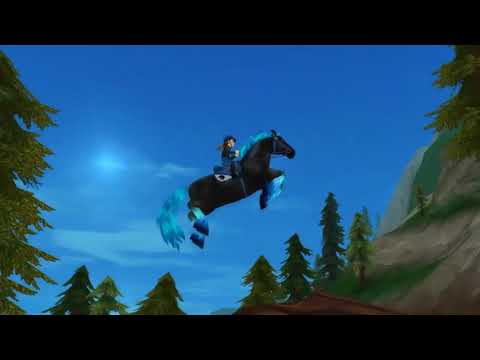This vibrant image, reminiscent of a screen grab from a video game or a charming cartoon, showcases a dynamic scene framed by horizontal black letterbox borders. The background features a blue sky accented with a few clouds and the faint hint of a sun, which illuminates a lush landscape dotted with evergreen trees. These trees appear on both the left and right sides, partially cut off by the image frame, and cascade down a hillside into a brown plateau.

Dominating the center of the image is a striking black horse mid-air, creating an illusion of flight. This fantastical creature has distinctive blue accents on its mane, tail, legs, and hoofs. Astride the horse is a person, possibly a little girl dressed in equestrian gear, evoking a whimsical, storybook feel. The horse appears to be soaring over the sloped terrain below, adding to the sense of adventure and magic captured in this enchanting scene.